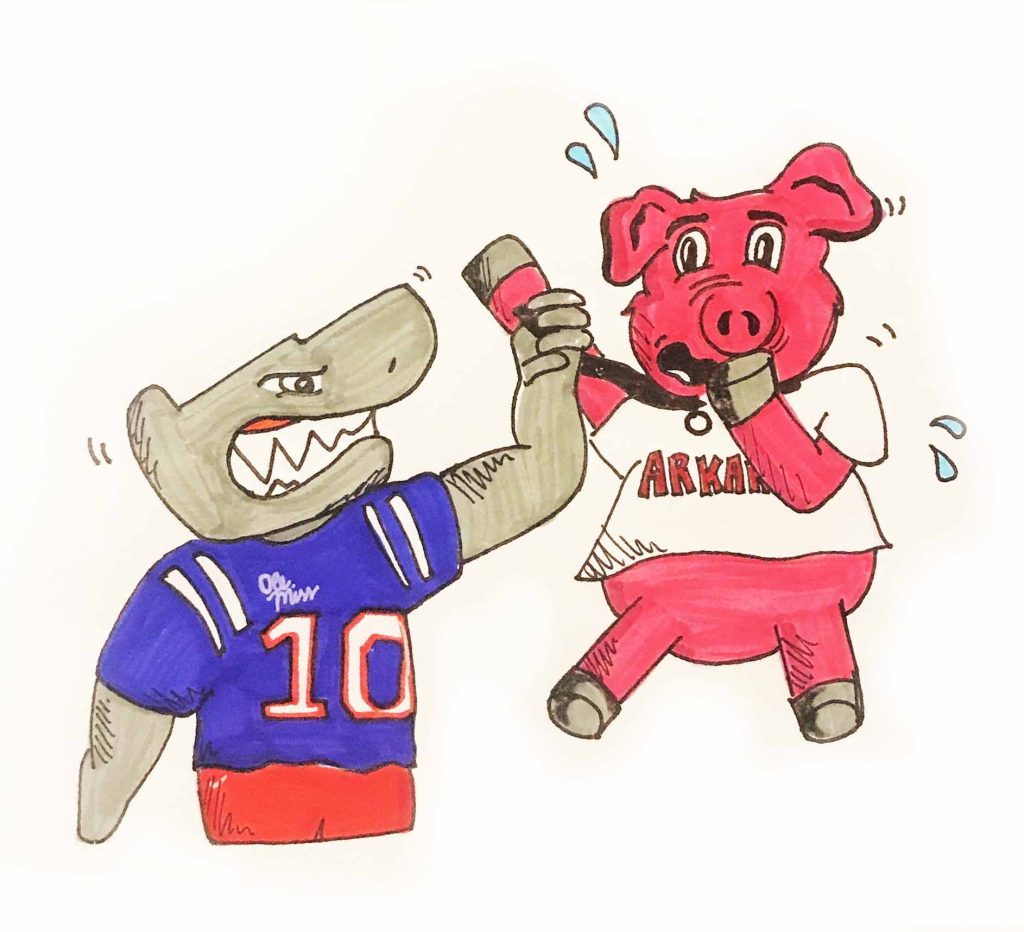This lively cartoon illustration features a dramatic scene between two anthropomorphic characters: an aggressive shark and a frightened pig. The shark, positioned on the left, stands dominantly and appears menacing with an enraged expression. It is drawn in shades of green and sports a blue jersey emblazoned with "Ole Miss" in white cursive and the number 10 outlined in red. The jersey has white shoulder stripes, and the shark completes its intimidating attire with red shorts cut off at the upper thigh. The shark is gripping the necktie or collar of the pig, which adds to the tension of the scene.

The pig, on the right, is vividly colored in dark pink and wears a shirt that reads "Arkansas." It has no pants. The pig’s face is contorted in terror, with wide eyes and its mouth partially covered by one hoof, which also reveals an open mouth. Sweat droplets and lines indicating shaking surround the pig, emphasizing its fear. This detailed and energetic illustration captures a moment of intense confrontation, highlighting the contrasting emotions of the confident, aggressive shark and the scared, vulnerable pig.